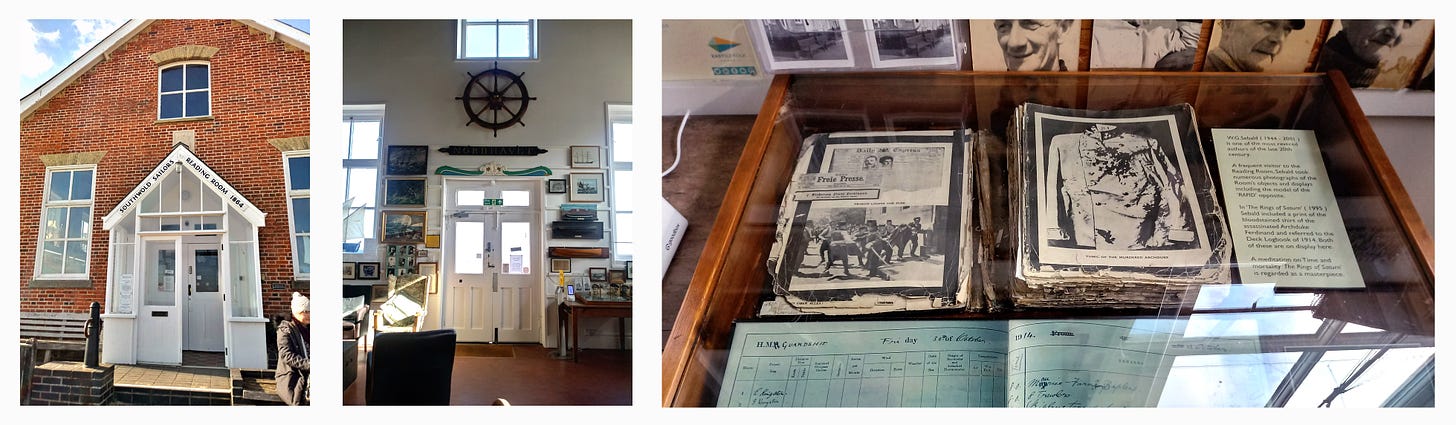This collage of three horizontally aligned photographs creates a detailed visual narrative. On the left, an exterior shot captures a stately brick building with a white gazebo-style entrance, reminiscent of an old one-room schoolhouse, complete with large double doors and three sizable windows. The middle photograph transitions us to the interior of this building, revealing the same doorway from the opposite side. The inside showcases white walls, brown floors, and multiple frames on the walls, dominated by a large ship captain’s wheel mounted above the doorway. There are a few desks with old-fashioned lamps and scattered paperwork, giving a sense of clutter. The rightmost image focuses on a wooden glass-topped display case filled with vintage documents, ledgers, and black-and-white photographs, some of which are also visible on the wall behind the case. This series of images offers a rich, detailed glimpse into a historic setting, blending architectural elements with maritime memorabilia and historical records.